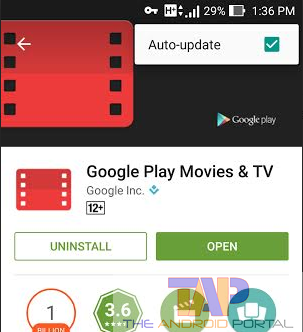**Caption:**

A cropped screenshot of an Android phone, showcasing the middle and upper portions of the screen. The interface is centered towards the right, displaying various app icons. Among these icons, there's an image of a key and a white square containing an "H" symbol, accompanied by up and down arrows. Bars for cell phone signal strength are visible, indicating 29% completion. The battery icon and a clock showing 1:36 p.m. are also present.

The screen features a red movie reel icon with a back arrow on the left, next to a white rectangle with the text "Auto Update" in black. Adjacent to it is a turquoise square featuring a white checkmark. The background of this section is predominantly black, with "Google Play" text situated to the right.

Below the black section, the background switches to white, repeating the red movie reel icon. "Google Play Movies & TV" text appears next to it, followed by "Google and company." A logo and a "12+" age rating in a box are visible. Two buttons underneath offer options to "Uninstall" and "Open" the app.

Lower on the screen, there are various additional buttons: a red circle with a "1" inside, a green stop sign-shaped button indicating a rating of "3.6" stars, and two other unspecified icons.